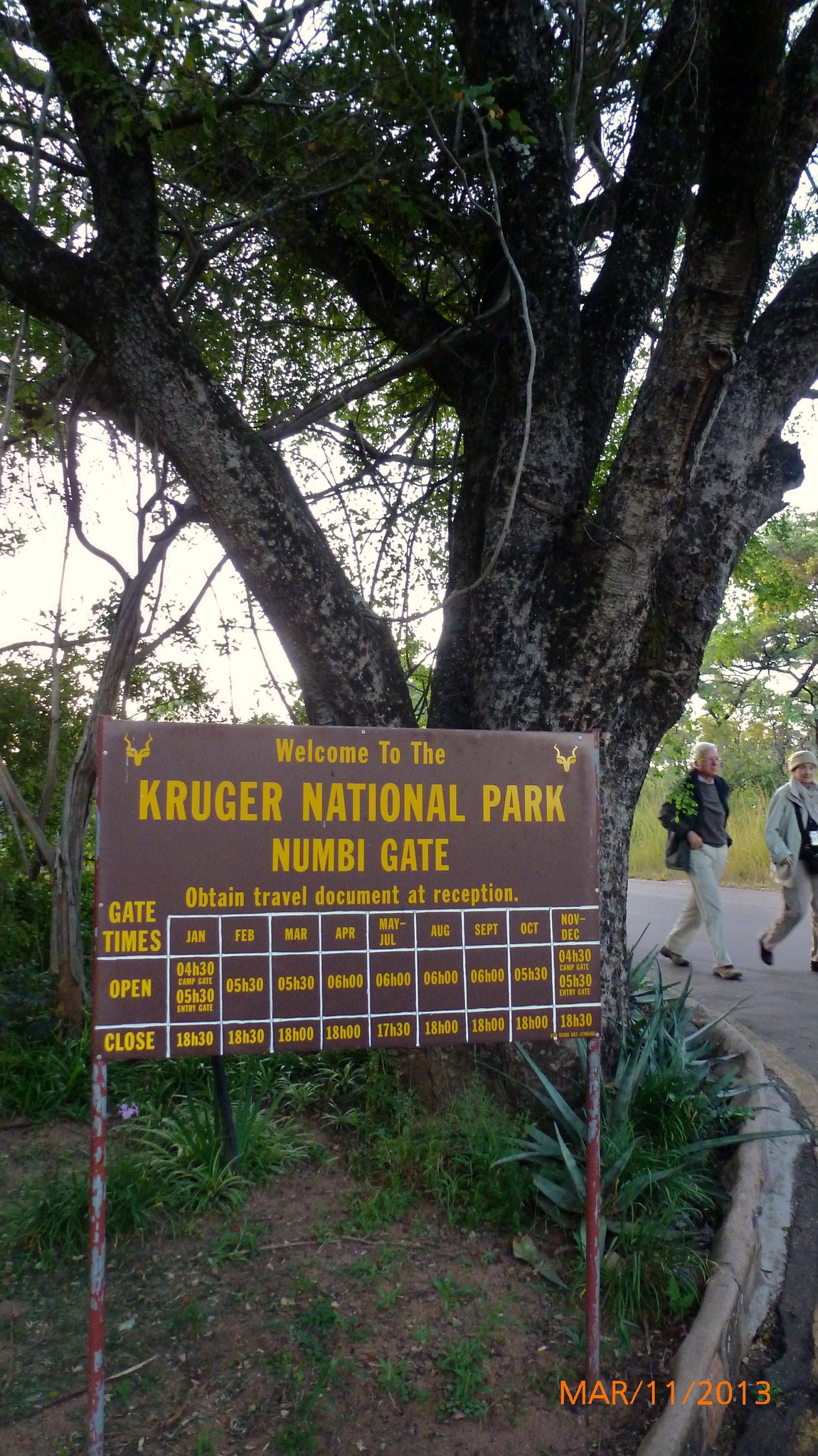In the foreground of this overcast yet sunny March 11, 2013, photograph stands a prominent brown sign supported by two weathered metal posts, embedded in a concrete-curbed median adorned with a variety of plants including aloe-like vegetation. The sign, welcoming visitors to the Kruger National Park at Numbi Gate, provides crucial information: "Obtain travel document at reception" and lists gate times alongside the respective opening and closing hours, categorized by months. To the right of the sign, an expansive grass field stretches into the background, bordered by a large, dominant tree. In the midground, two older individuals are captured walking along the park's pathway—one in a black shirt with white pants, the other in a white jacket and tan pants—adding a sense of scale and life to the serene park environment.